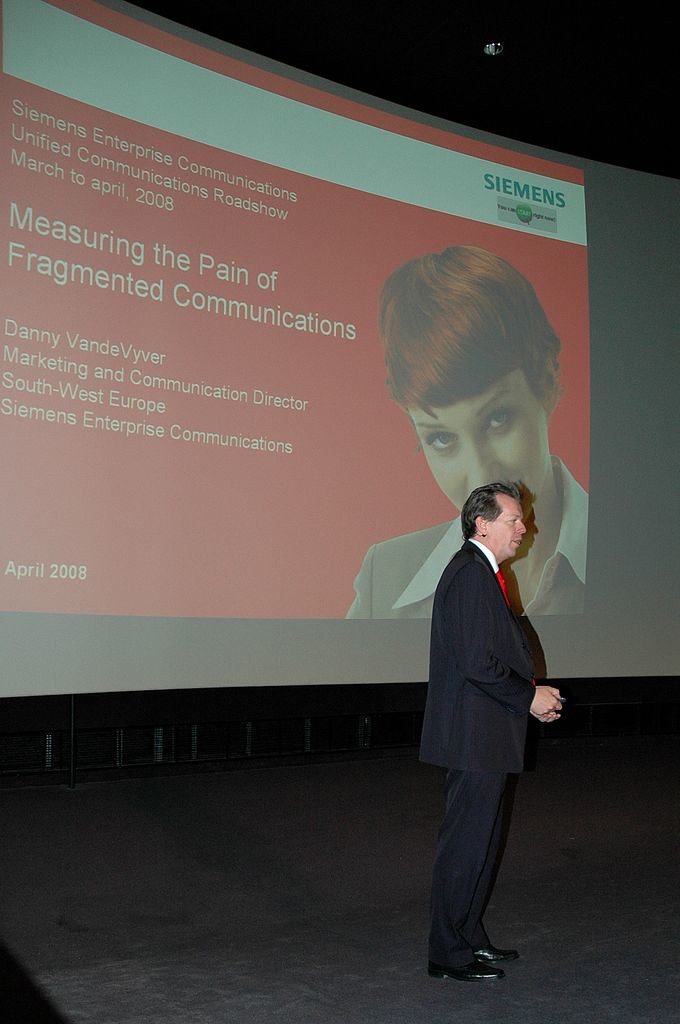The image captures a middle-aged man with black hair, dressed in a black suit, white shirt, and red tie, standing sideways on a dark stage. He is illuminated and seemingly engaged in delivering a lecture. Behind him, there is a brightly lit slide projected on a screen that bears the title "Measuring the Pain of Fragmented Communications." The slide features a red background with white text, and includes an image of a woman in the lower corner. Further details indicate that this is part of the Siemens Enterprise Communications Unified Communications Roadshow, dated March to April 2008. The text also lists the role and name of Danny Venn, Director of Marketing and Communications for Southeast Europe, highlighting the conference's focus on communication challenges.